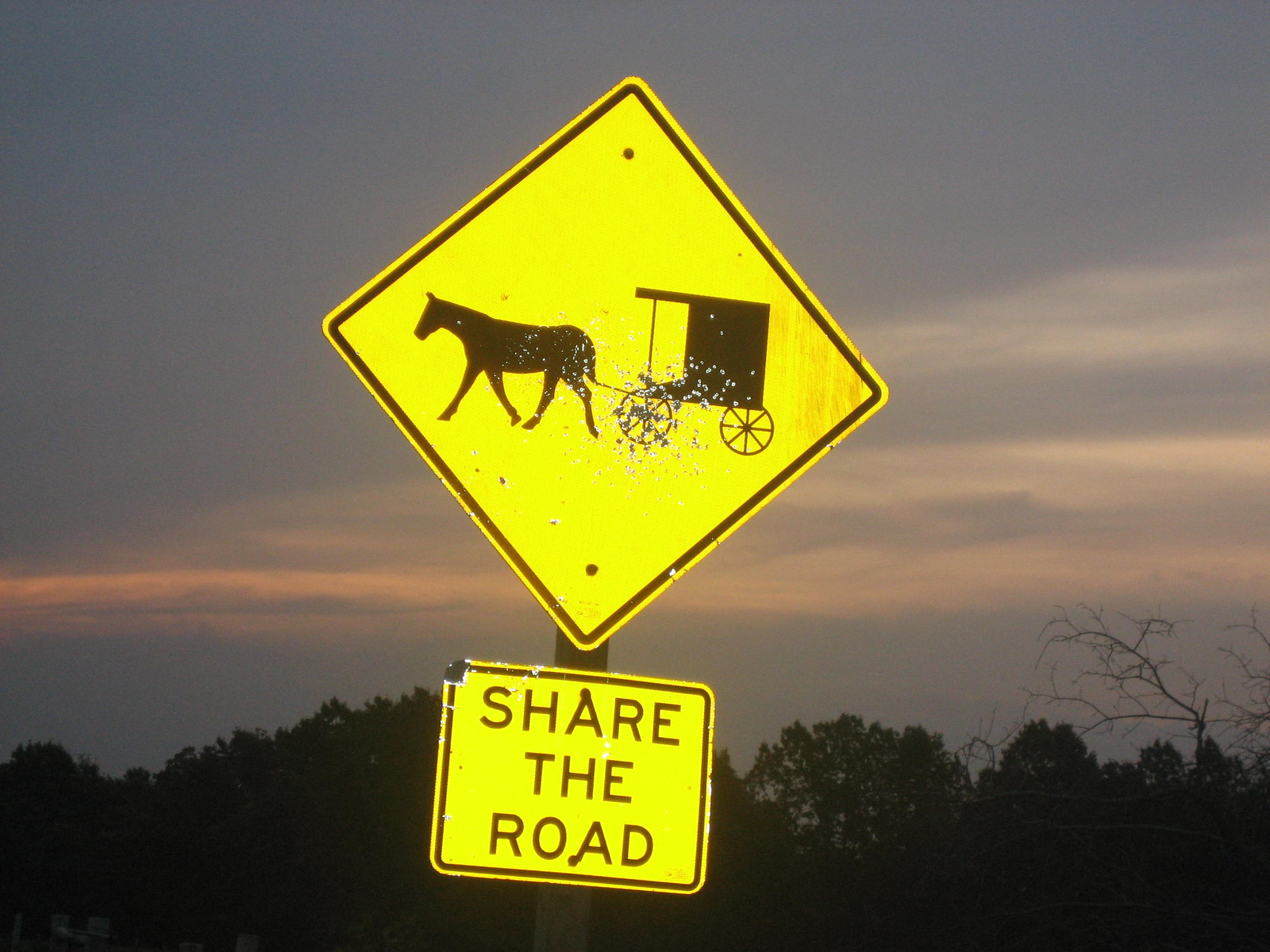This photograph portrays a road sign cautioning for horse-drawn buggies with a directive to "Share the Road" displayed below. Mounted on a single post in the center, the top sign is a bright yellow diamond with a black silhouette of a horse pulling an Amish buggy, depicted with rudimentary details. Below it, a square neon yellow sign with black lettering reiterates to "Share the Road." Both signs exhibit reflective qualities, although the top sign is pocked with numerous defects, likely from BB gun or shotgun pellets. The backdrop features a dense array of tall trees, predominantly vegetative, except for one towering, leafless tree on the far right. The sky suggests either dawn or dusk, showcasing a gradient of dark blue, purple, and red hues with streaks of clouds enhancing the serene yet somber atmosphere.